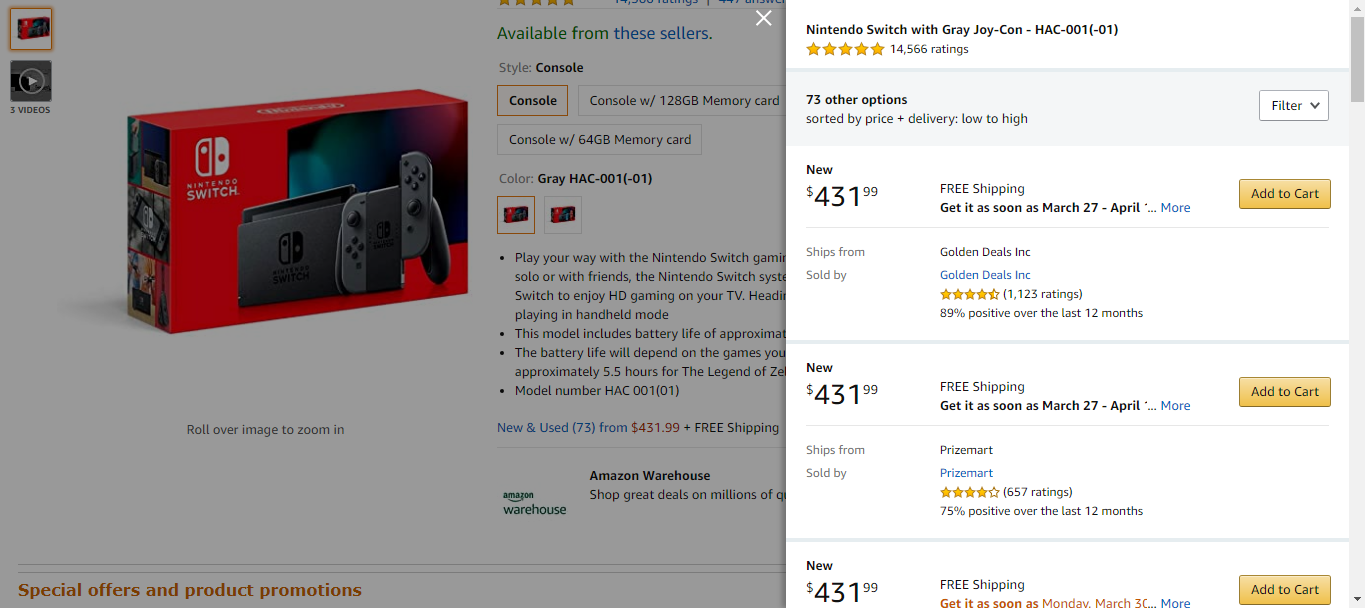The image features a Nintendo Switch product showcased on an Amazon product page. On the left side of the page, there is a large image of the Nintendo Switch console's packaging box. The box is primarily red and prominently displays the Nintendo branding. The box is angled such that the front of the box is slightly facing to the right.

The style of the product is specified as a console, and the color of the console is gray. The model number HAC-001 (also listed as HAC-001(-01)) is noted on the packaging.

On the right side of the page, there is a brighter section featuring pricing information. This section is divided into three rows, each displaying the same price for a new Nintendo Switch console, listed at $431.99.